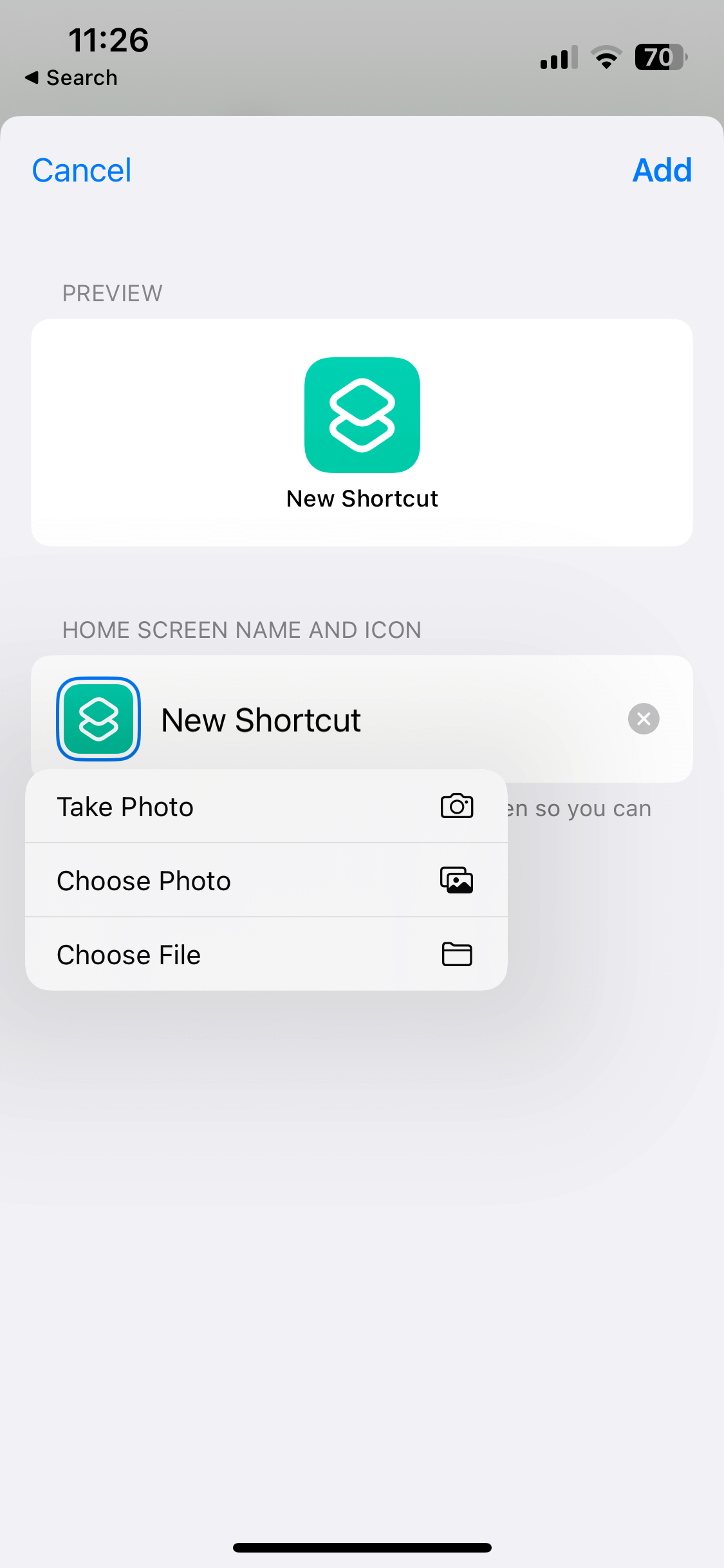This screenshot displays a variety of details on an iPhone interface. In the top left corner, the time is shown as 11:26. Adjacent to this, in the top right corner, the network signal bar indicates 3 out of 4 bars of signal strength. Next to it, the WiFi signal icon shows a connectivity strength of 2 out of 3 bars. The battery level is at 70%. Also in the top corners, the 'Cancel' option is located on the left, while the 'Add' option is on the right. The main section of the screen displays a preview for creating a new shortcut, titled "New Shortcut." Below this title, there are options for selecting a home screen name and icon. Further options include "Take Photo," "Choose Photo," and "Choose File," listed in a vertical arrangement. The background of the interface is white, enhancing the visibility of the text and icons. At the bottom of the screen, the standard black navigation key of the iPhone is visible.